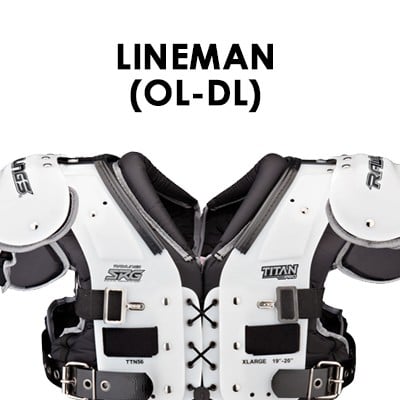This photograph displays a pair of black and white protective football shoulder pads, commonly used in American football. The outer shell is composed of bright white hard plastic, while the interior features softer black cushioning. Various adjustment straps are present, including thicker black leather straps with silver buckles towards the bottom, designed to secure around the lower chest. Black text on the shoulders and chest includes the brand name "Titan" on the left chest and "SRG" on the right. The shoulder pads are marked with text at the top of the image, indicating their use for linemen, specifically for Offensive Line (OL) and Defensive Line (DL) positions.